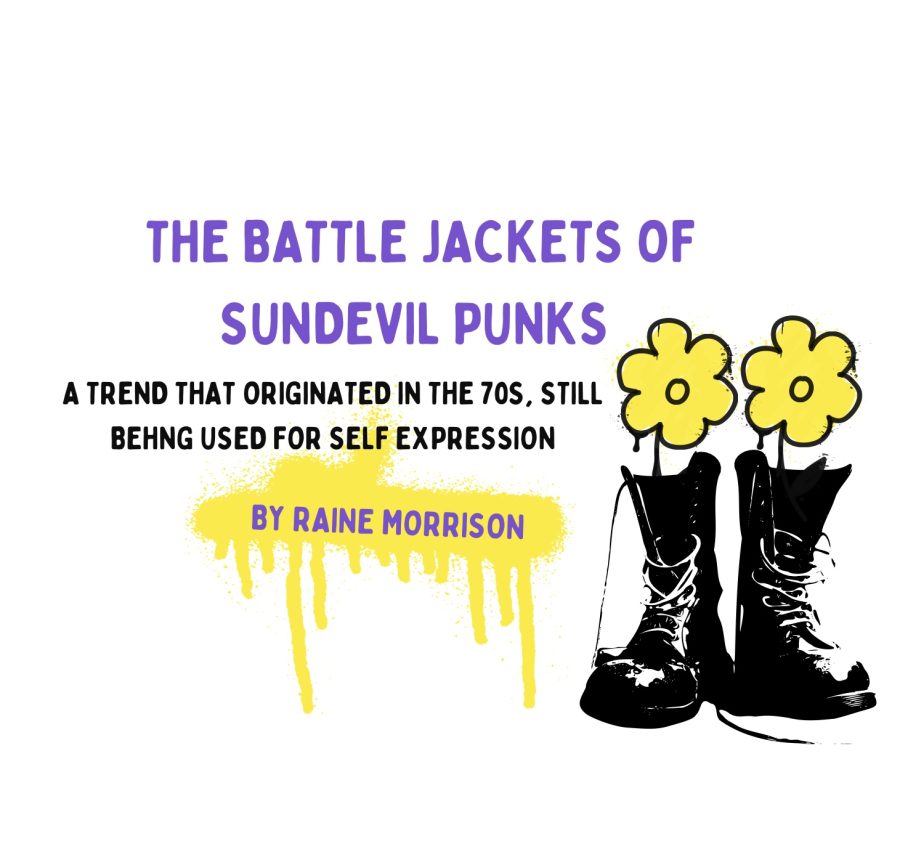The image appears to be a computer-generated cover art featuring a bold, all-caps title in bright purple text positioned centrally, which reads "THE BATTLE JACKETS OF SUN DEVIL PUNKS." Beneath the main title, smaller bold black text states, "A TREND THAT ORIGINATED IN THE 70S, STILL BEING USED FOR SELF-EXPRESSION." A diagonal spray paint line, in yellow and dripping downward, runs across the image, and inside this line is purple text that identifies the artist: "BY RAIN MORRISON." To the right of the text, there is a pair of black combat boots with white laces, each boot having a sketchy yellow flower growing out from it. The background of the image is entirely white.